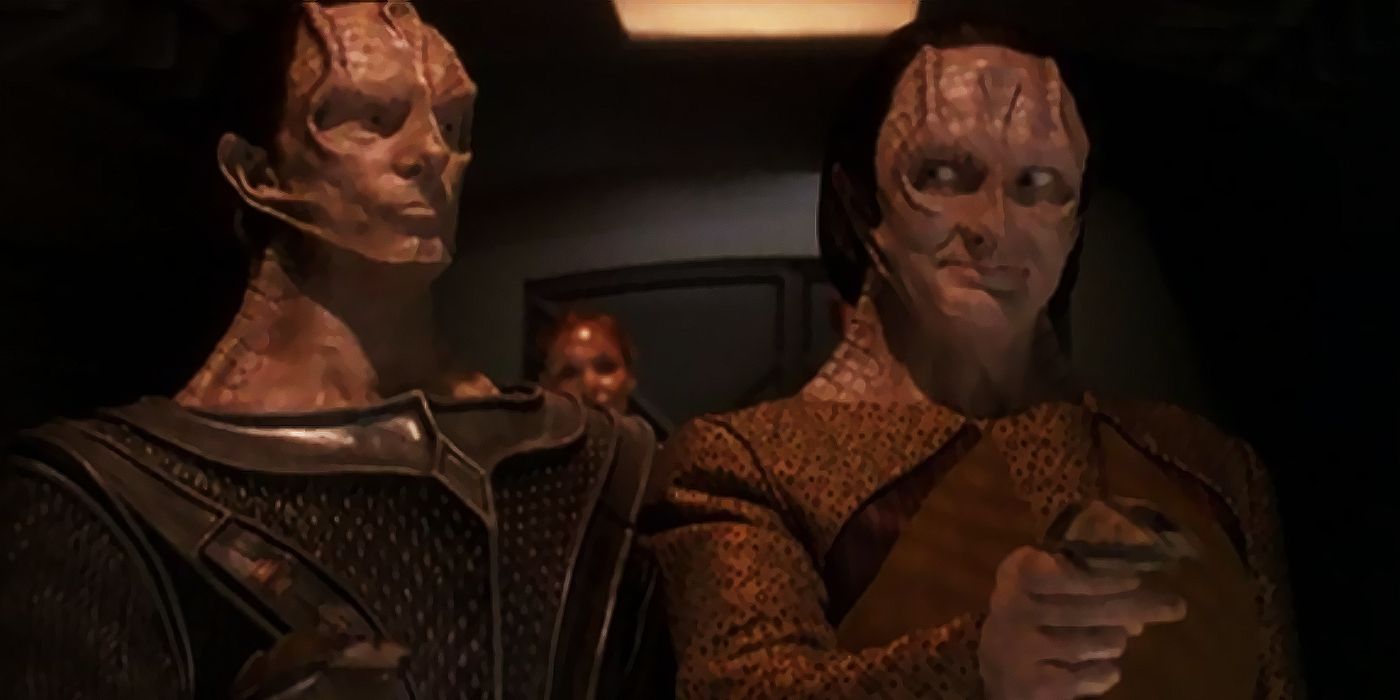In this image, we see a scene that appears to be from a science fiction TV show. The central focus is on two humanoid figures with alien-like, scaly, white, lizard-like skin and thick necks. They both wear long-sleeve, bronze-colored uniforms that resemble armor. Their heads are distinctively characterized by raised foreheads and blank eyes. The figure on the left seems static, while the one on the right is more dynamic, holding an angled, weapon-like device with an extended right arm. In the background, a startled human-looking woman peeks into the room over their shoulders. All three characters stand in front of a door illuminated by a red fluorescent light at the top edge.